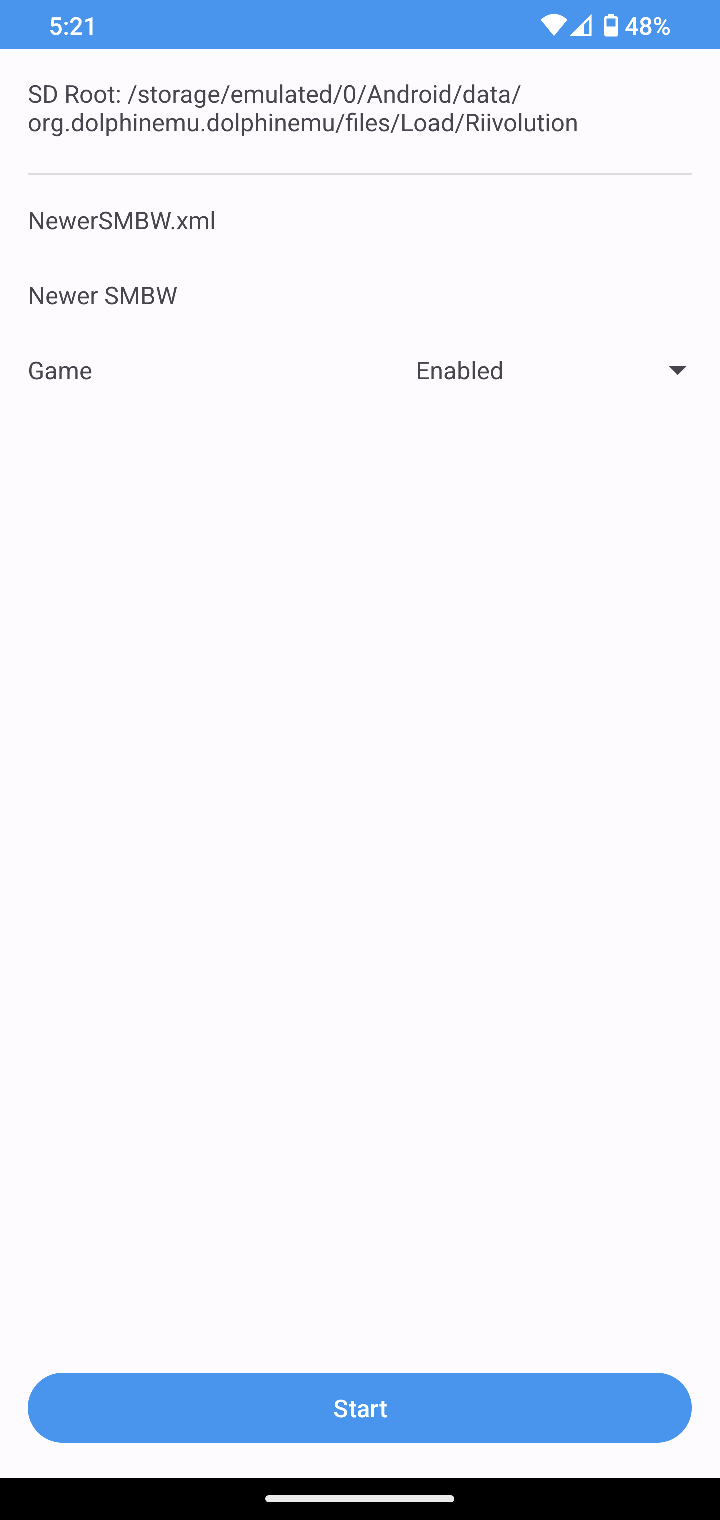The image appears to be a screenshot taken from a smartphone. At the top, the status bar displays the time as 5:21, with various icons indicating a strong Wi-Fi connection and a battery level at 48%. Below the status bar, there is a navigation path that reads: "sd root / storage / emulated / 0 / android / data / org.dolphinemu.dolphin / files / load / revolution." This path is followed by three columns labeled: "newer_smw.xml," "newer_smw," and "game."

The "game" option in the third column is currently set to "enabled," suggesting it can be toggled between enabled and disabled settings. Toward the bottom of the screen, there is a prominent blue button labeled "Start." Beneath this button is a black rectangle with a thin white line running horizontally through its center. The overall layout and design suggest the interface of an application, possibly the Dolphin Emulator, used for managing and launching games.